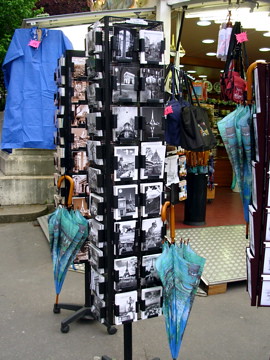The image showcases a tall, spinning card holder display stand situated outside a storefront. The primary stand features an array of eight black-and-white photos arranged in two vertical rows of four, creating a visually appealing column. Hanging from this stand are umbrellas with brown handles and blue canopies, reminiscent of ocean or sky motifs. In the background, another similar card holder with an umbrella is visible, and further to the left, a third stand with part of another umbrella can be seen at the edge of the photo. Behind these displays, a blue shirt or dress with a pink price tag is prominently featured, with other indistinct items providing a hint of the store’s assortment. The ground appears to be asphalt or concrete, suggesting an outdoor setting, further hinted at by the subtle presence of what looks like a tree in the top left corner of the image.